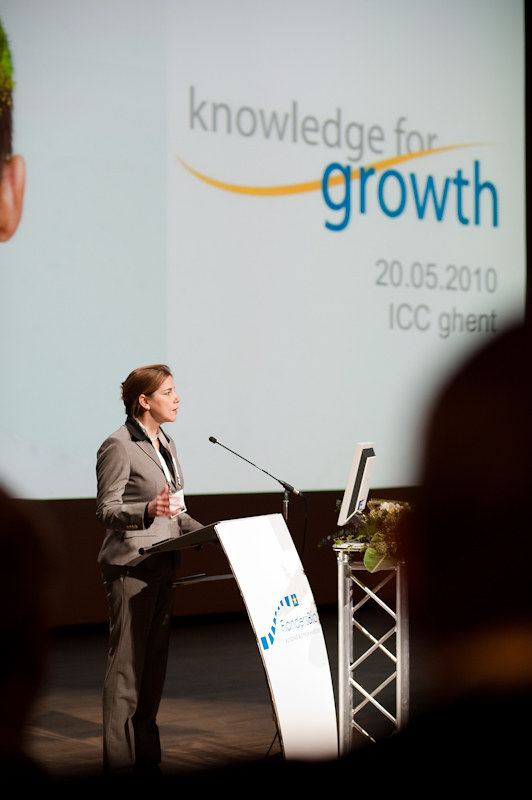In this tall, rectangular image, a woman is seen giving a presentation at a podium positioned on the left side. The woman, who has short brown hair tucked behind her ears, is dressed in a beige-gray suit and is visible from her feet up. The podium has a white and blue advertisement panel on its front, and she's speaking into a slender microphone extending from the podium. The background features a very large screen displaying an advertisement with the words "Knowledge for Growth," where "Knowledge" and "for" are in gray and "Growth" is in blue, accompanied by a yellow swirly line. Below this, the text reads in gray, "2005-2010, ICC Ghent." The stage is dimly lit, but the top area is well-illuminated. In the bottom right corner, there's a blurry silhouette of a man's head, and a few other out-of-focus heads are visible, highlighting the audience.